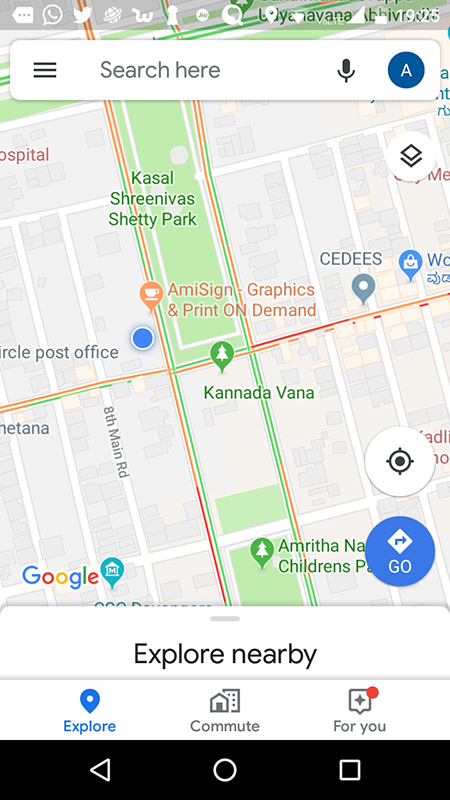**Detailed Caption for the Image:**

The image is a screenshot from an Android smartphone, depicting a Google Maps interface captured at 19:25. At the top of the screen, several notification icons are visible, including WhatsApp, Twitter, and the Google system notifications, indicating the phone is connected to a high signal with a moderate battery level. 

The Google Maps UI features a search bar at the top labeled ‘Search here’ by default, accompanied by a hamburger menu on the left, a microphone icon for voice search, and the account holder’s initial 'A' in a blue circle representing their Google account.

The map displayed includes various geographic and locational details. Notable landmarks include:

- A post office marked by a dot.
- “Amnesty and Graphics and Print On Demand” and a coffee shop icon.
- Green areas indicating parks, specifically Shetty Park and Amrita Children's Park.
- Street names such as Kaysfield Street and Kanata Vanna.
- A partly visible hospital located in the top left corner.

Several light gray buildings signify other public or residential buildings. Additionally, a ‘campus’ is identified on the map, alongside options like “Explore Nearby,” “Explore,” “Commute,” and “For You” with personalized recommendations at the bottom of the interface.

Other visible icons include the ‘ghost option’ (potentially an incognito mode), the Google logo, and a partial label identifying Leicester Financial Institution.

This detailed description captures the comprehensive layout and notable features presented in the Google Maps screenshot on an Android device.